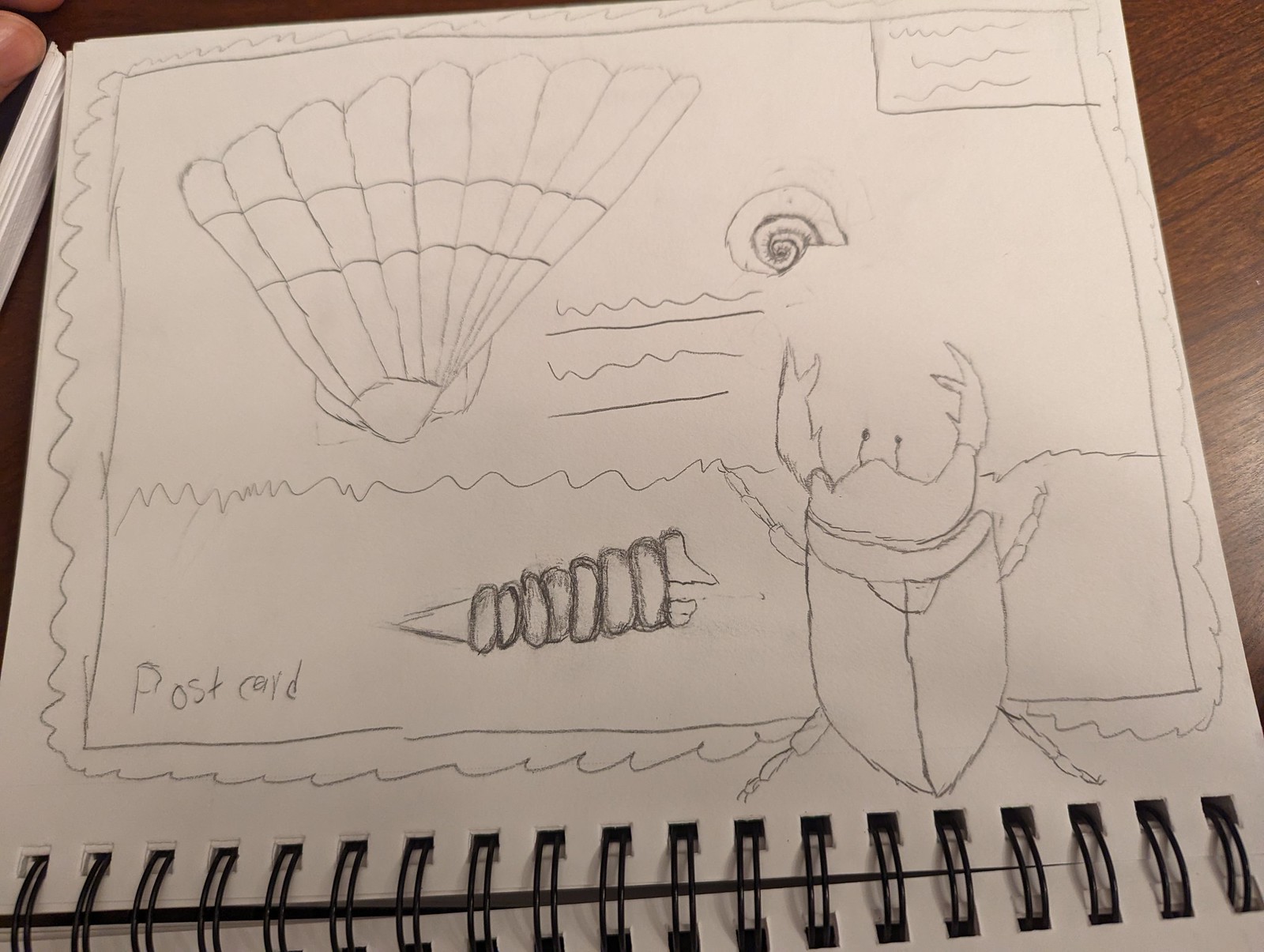This photograph captures a sketchbook open to a page showcasing a detailed pencil sketch. The spiral binding of the sketchbook is visible at the bottom of the image. The sketch on the page resembles a frame of a postcard, with "Postcard" inscribed in the bottom left corner. Dominating the illustration are various beach-themed elements: a large fan-like shell, a spiral shell resembling a nautilus, and another shell with a more snail-like appearance. Additionally, there's a rectangular area intended to represent a stamp. A significant portion of the sketch is occupied by a large beetle-like creature, though it only has two legs, which contrasts with the six legs typically associated with insects. The sketch captures the essence of seaside treasures and combines them into a whimsical, postcard-themed illustration.